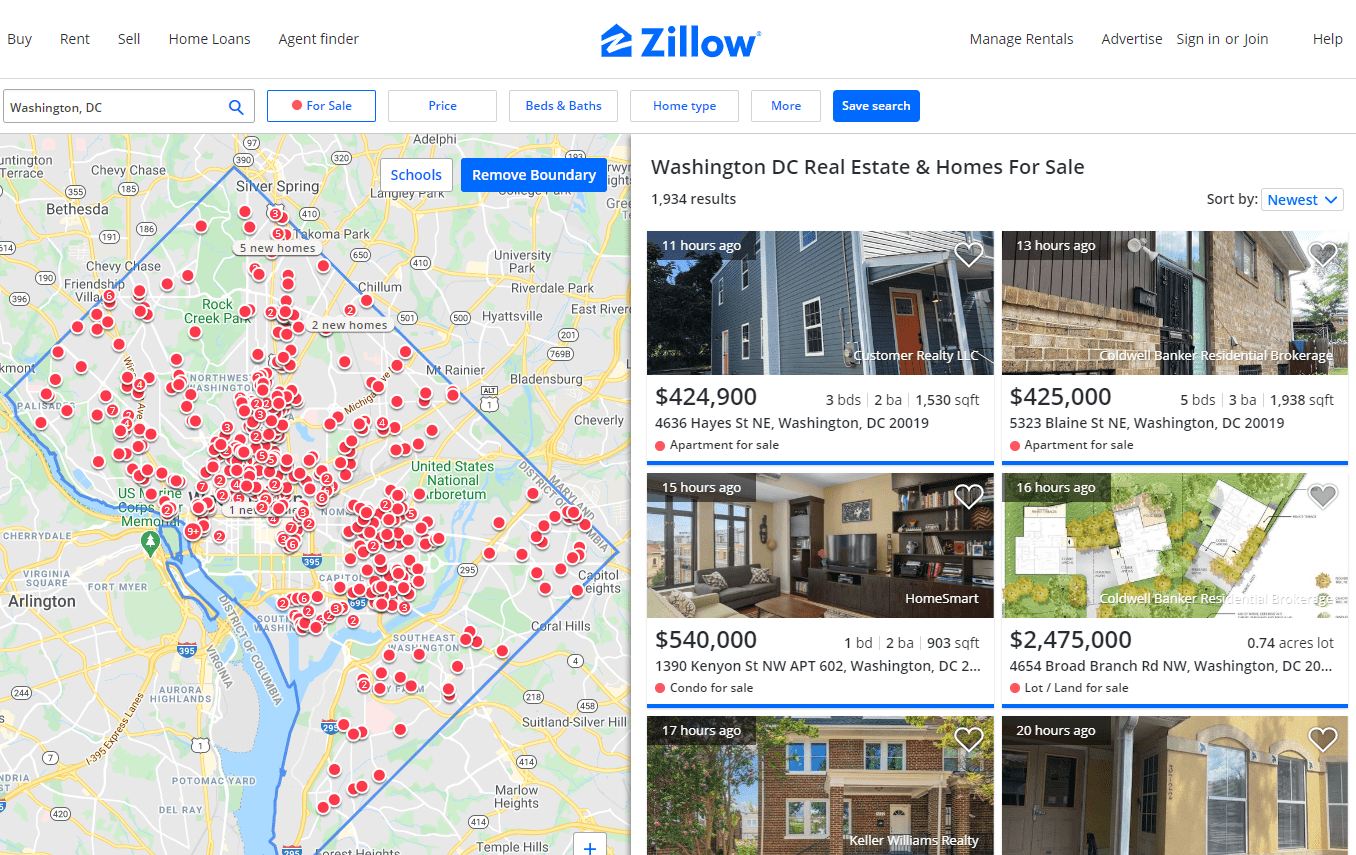This screenshot of the Zillow homepage showcases its user interface in meticulous detail. The Zillow logo is prominently positioned at the top center. To the upper left of the logo is a horizontal menu, mirrored by another horizontal menu on the upper right side. Directly beneath the Zillow logo is a search bar, which includes several filtering options, starting from left to right: a search bar, a "For Sale" button, a "Price" button, a "Beds and Baths" button, a "Home Type" button, and a "More" button. The search functionalities are completed with a "Save Search" button.

On the left side of the screenshot below these elements is a map, while on the right side are the search results displayed as property listings. The right-hand section features six property images, arranged in two columns and three rows, each labeled with "Washington, D.C., real estate and homes for sale" and sorted by "Newest."